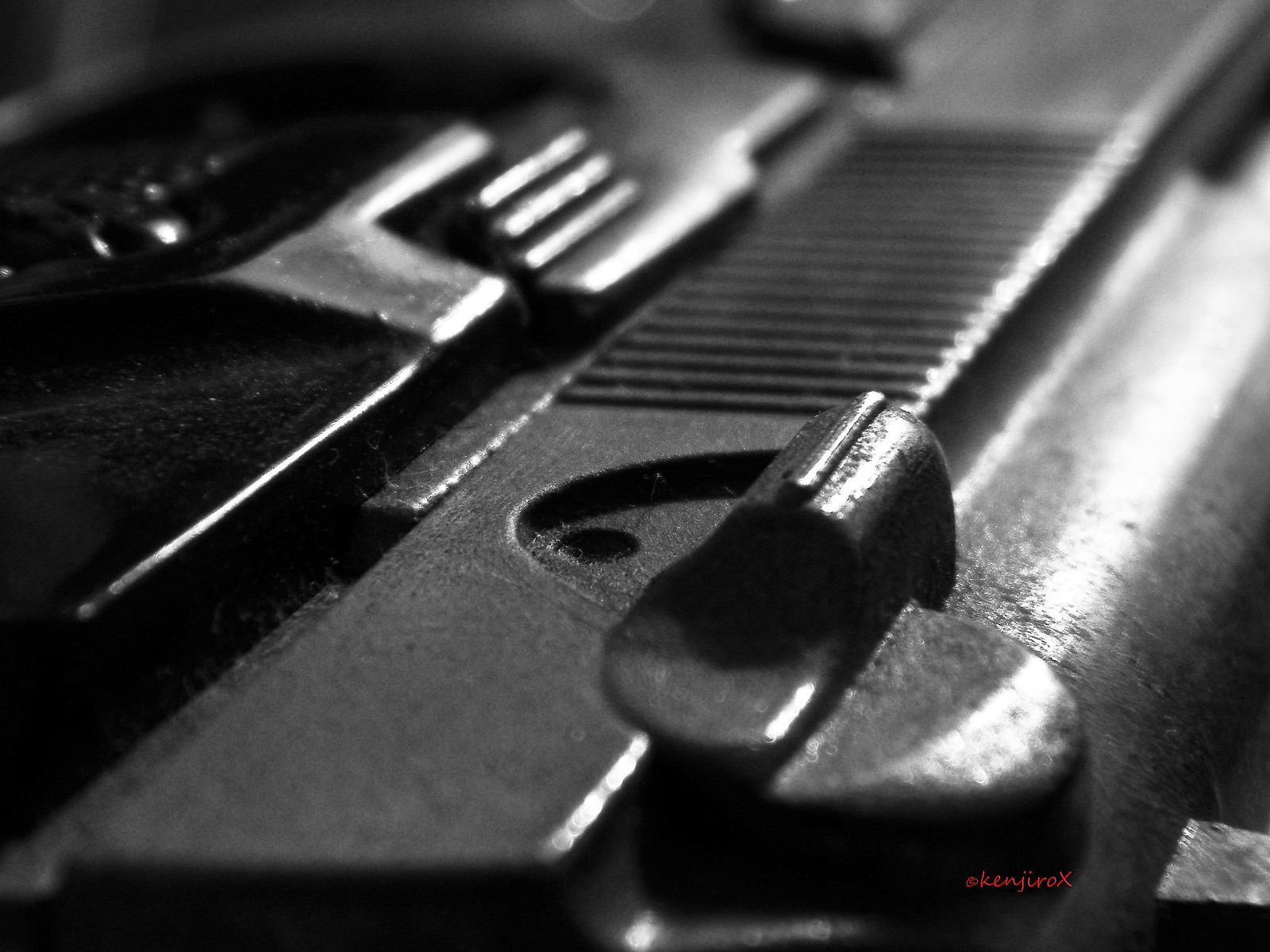This image is an extremely close-up photograph of what appears to be a black metallic gun, specifically focused on parts of the barrel and trigger region. The photograph, taken in landscape orientation, only captures about three or four inches of the gun, making it difficult to identify specific model details. The image highlights the locking mechanism and the trigger area, where intricate details such as where the finger would go can be seen. The surface of the gun shows a mix of matte and glossy finishes, with a light source creating a shine on the upper right area. Notably, at the bottom right in red text, it reads "KENJIROX." This detailed close-up emphasizes the metallic texture and components, providing just enough information to suggest it's a pistol.